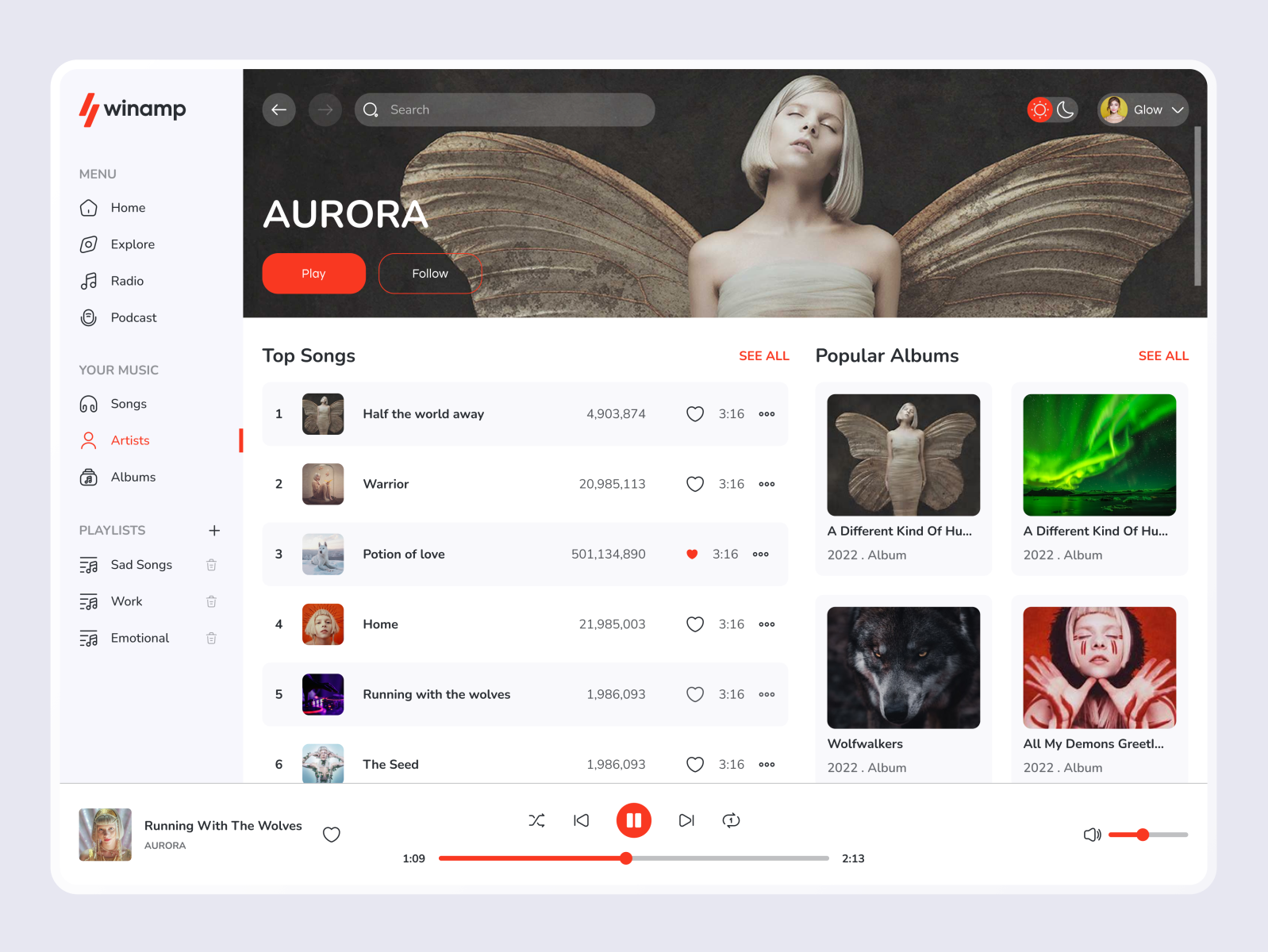On the displayed website, the side panel features the name of the application, WinAmp, prominently at the top. Below the application name is a menu categorized under different headings. The first heading, "Menu," includes options such as Home, Explore, Radio, and Podcast. The next heading, "Your Music," lists categories like Songs, Artists—currently highlighted in red—and Albums. The final heading, "Playlists," showcases various playlist names, such as Sad Songs, Work, and Emotional.

The main screen showcases a striking banner featuring a woman with a blonde bob haircut up to her shoulders, adorned with moth-like wings, and bandages across her chest. The banner introduces the artist, Aurora, with a red-highlighted "Play" button. Beneath the banner is a list of top songs, numbered one to six: Half the World Away, Warrior, Potion of Love, Home, Running with the Wolves, and The Seed.

To the right, there's a section titled "Popular Albums," displaying four small thumbnails of album cover artwork, adding a visual element to the user interface.